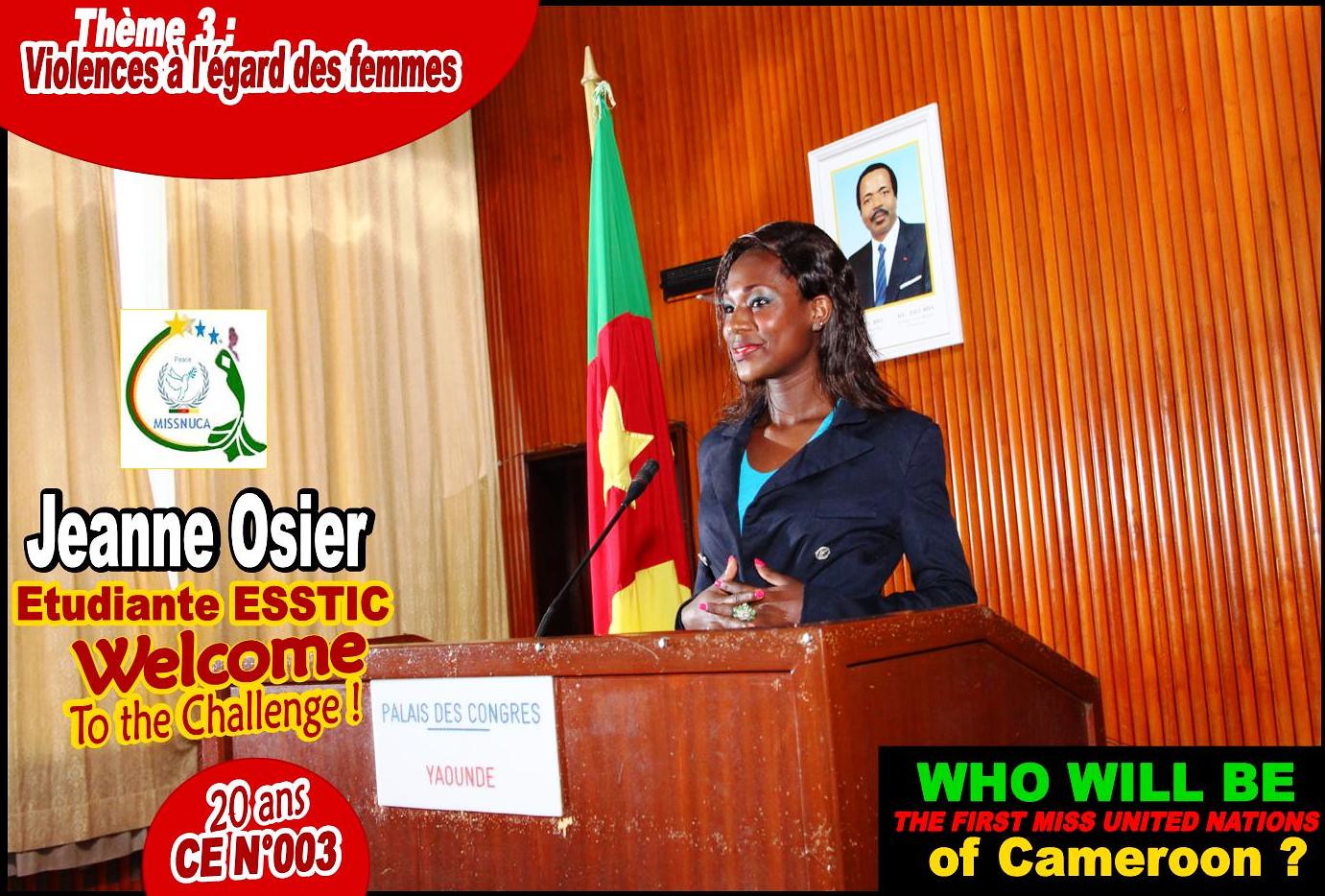In the center of the image stands a woman at a wooden podium, speaking into a microphone that points directly at her face. To the left of her, a national flag is prominently displayed. The podium is positioned against a backdrop of a wooden wall, with a curtain on the left side partially covering a window. The wall and curtain create an indoor setting, suggesting the event is taking place during a press conference. The podium bears text in a different language, with the readable portions stating "Jean Ossier. Welcome to the challenge. Who will be the first Miss United Nations of Cameroon?" The image features a vivid array of colors, including brown, white, tan, black, dark blue, light blue, green, red, and yellow, adding to the dynamic atmosphere of the scene.